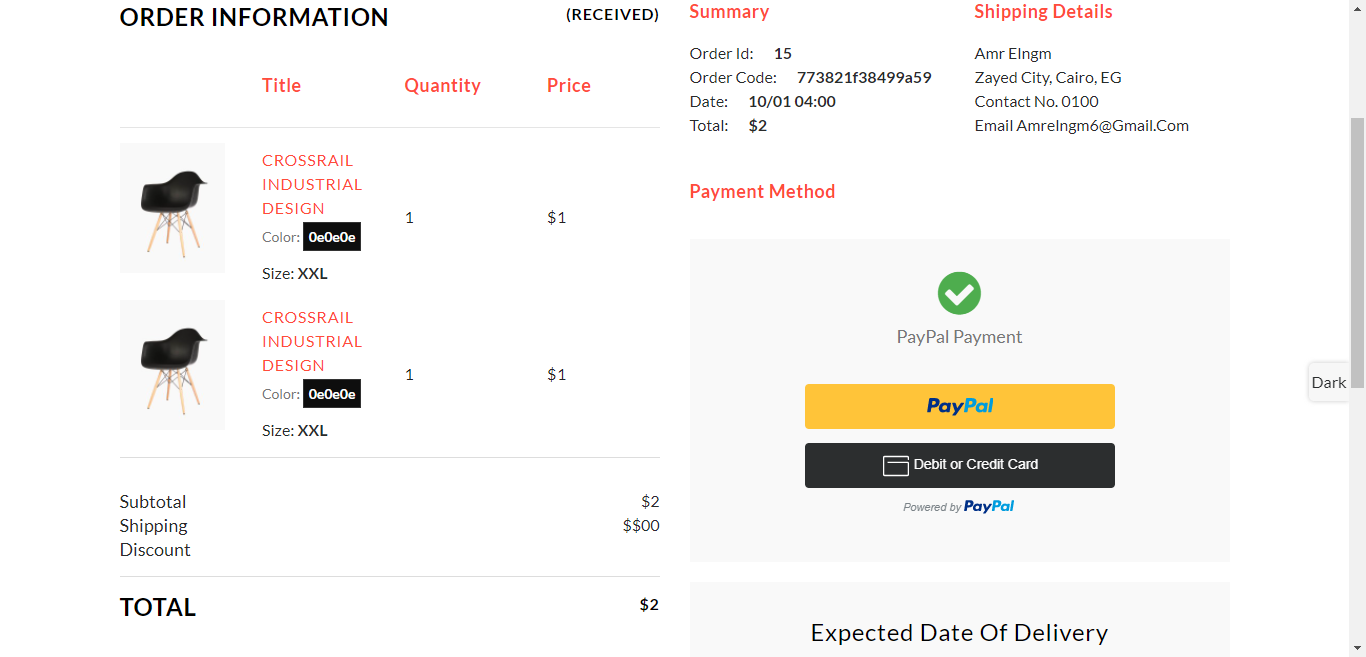Here is a detailed and cleaned-up caption for the given image:

"This screenshot from an unidentified website displays detailed order information. On the left, a vertical section itemizes 'Order Information', listing headings such as 'Received', 'Title', 'Quantity', and 'Price'. A photograph of a black chair with wooden legs is prominently featured. Adjacent to the image, the details reveal the chair's design as 'Crossrail Industrial', with a color code of 'OEOEOE', in size XXL. The listing specifies a quantity of 1, priced at $1 each. This same information is repeated below a second photograph of the chair. 

Further down, a breakdown of costs shows a subtotal of $2, zero shipping cost, and a discount totaling $2, effectively bringing the net price to zero. To the right, a summary provides the order ID '15' and order code '773821', with a secondary code 'F38499A59'. The order date is recorded as '10/1' at '4:00'. The total amount is listed as $2, with shipping details addressed to 'AMRELNGM, Zayed City, Cairo, Egypt'. A contact number '0100' and email 'AMREINGM6@gmail.com' are provided. The payment method is tagged as 'PayPal', specifying the use of PayPal debit or credit card. The expected delivery date information is partially cut off at the bottom edge of the image. The image does not feature any people."